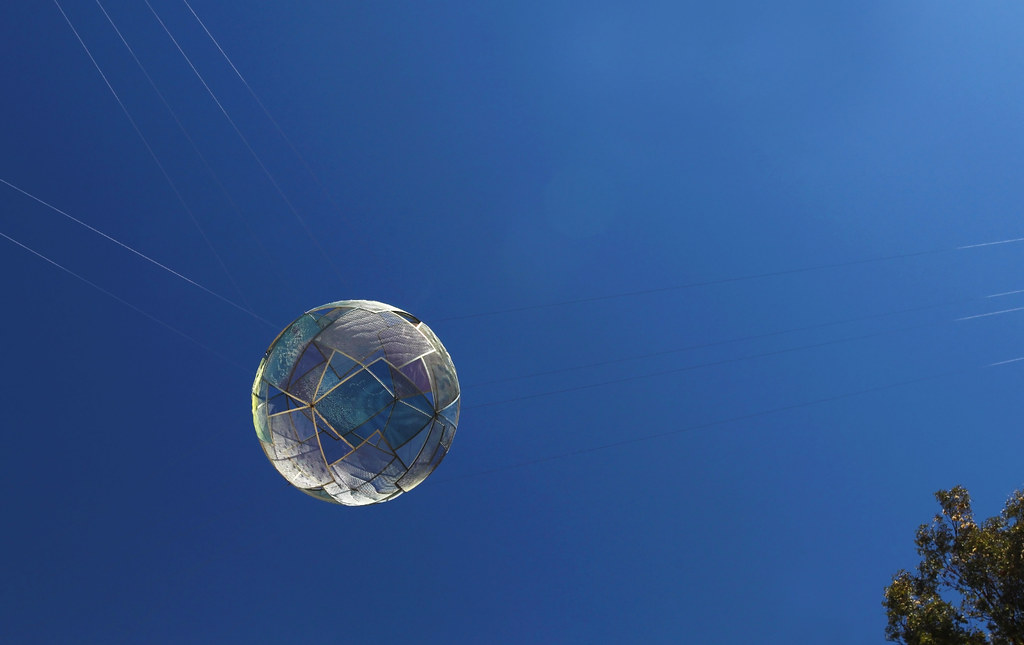The image captures a bright, cloudless blue sky with a tree's leafy branches in the bottom-right corner. Suspended in midair is a captivating artistic glass ball, held in place by several visible fishing lines converging at multiple points. The ball features intricate patterns of gold lines and purple shapes bordered in gold, reminiscent of stained glass. It's a striking piece of artwork that appears to glow in the sunlight, with white rays or lines outlining it against the sky. The strings and the ball's elevated position suggest it is displayed outdoors, potentially in a park, museum, or school setting.